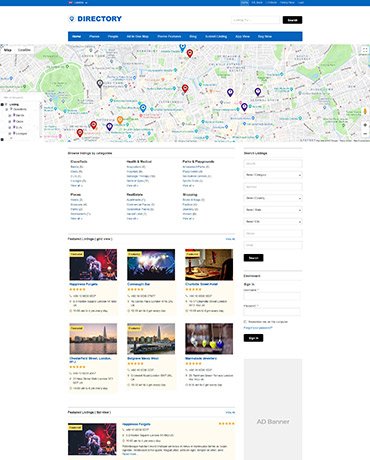This image features a digital directory interface. At the top, the word "Directory" is prominently displayed in blue, accompanied by a search bar positioned to its right. A thin blue strip runs along the very top, followed by a wider but shorter blue box below the directory title. Beneath this, there is a map dotted with small pins in red, purple, and blue, although the overall map is too miniature to discern specific details or locations.

Continuing downward, several categories are listed, each with headers in black and descriptive text in blue. To the right of these categories, there are drop-down boxes designed for information input.

Further down, the interface showcases a series of images that resemble covers or thumbnails. Two images display city scenes, one features a singer, another depicts a band with bright lights, and additional images include a desk setup and an arrangement that looks like balloons. Towards the bottom right corner, there is a photograph of a lone singer performing, accompanied by text about advertisements. This message is enclosed in a gray box labeled "AD BEGINNER."